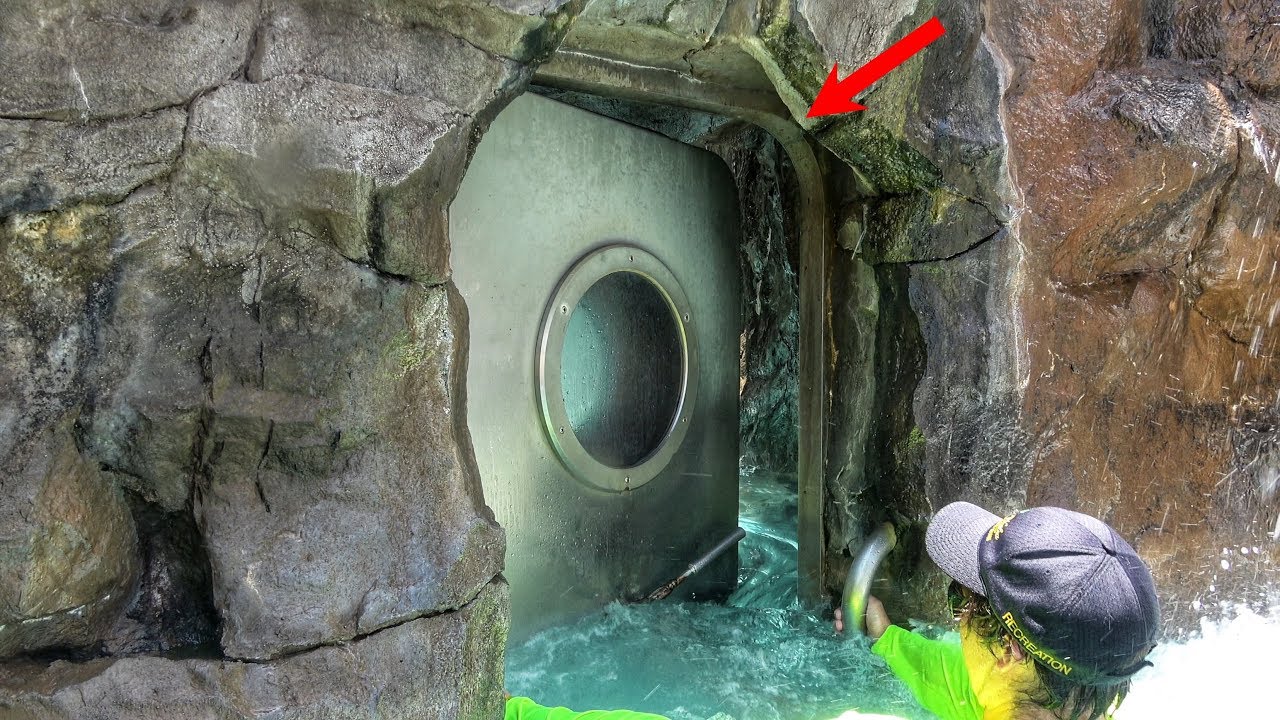The photograph, in a rectangular landscape orientation, features a captivating scene of a man chest-deep in rushing water. He is wearing a bright green shirt and a black baseball cap, and is positioned in the lower right corner of the image. The man grasps handlebars attached to a large, partially open metal door that’s set into a brown rock wall. The door, which is inundated by approximately four feet of water, has a large circular window or porthole in its upper portion. A red arrow is superimposed on the image, pointing downward toward the upper part of the door, adding to the visual intrigue. The door appears to lead into a water-filled passage, hinting at an extension of the rocky cave or structure beyond. No text accompanies the image.